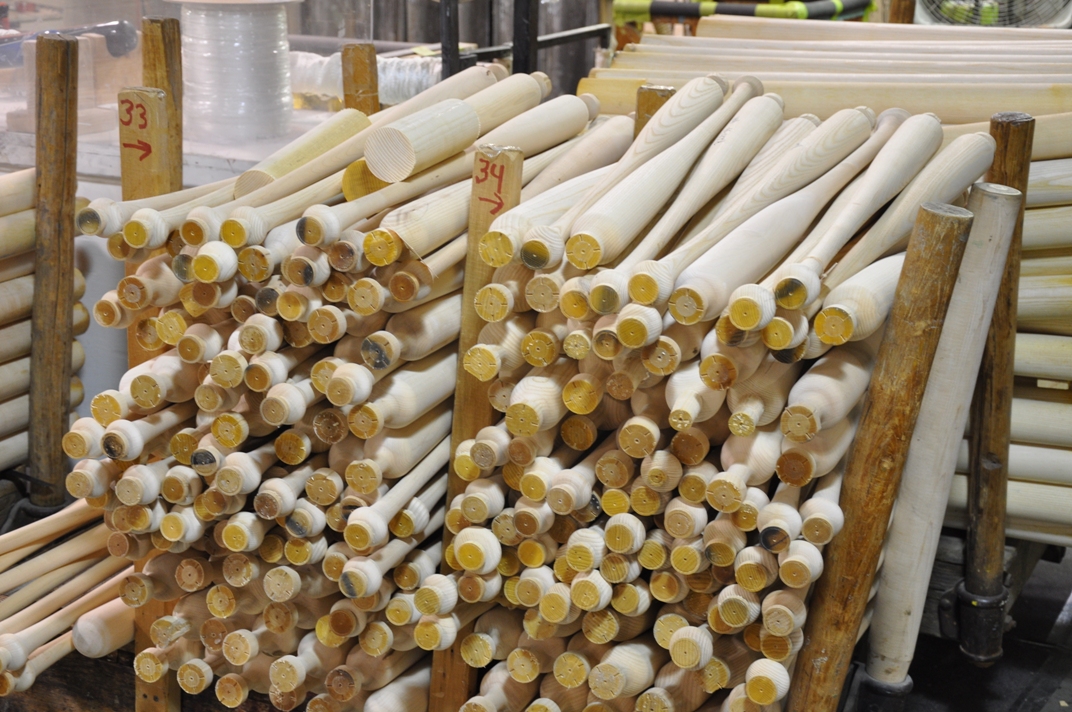The image depicts a bustling wood shop, likely a manufacturing facility, that specializes in creating table legs or similar shaped objects. Central to the image, you can see stacks of white wooden table legs with a distinct brown center, giving them a bordered appearance. These legs are piled in two separate groups, reminiscent of a scene with baseball bats due to their shape. One stack is labeled with '33' and an arrow pointing to the left, while another is marked '34' with an arrow pointing to the right. In the background, various shades of wood including dark browns are visible, adding depth to the scene. Additionally, there's a clear white cylinder present, surrounded by vertically stacked wooden planks. The wooden objects are numerous—potentially exceeding 200—and appear shaved down but not yet fully polished, highlighting the unfinished nature of the craftsmanship in progress.